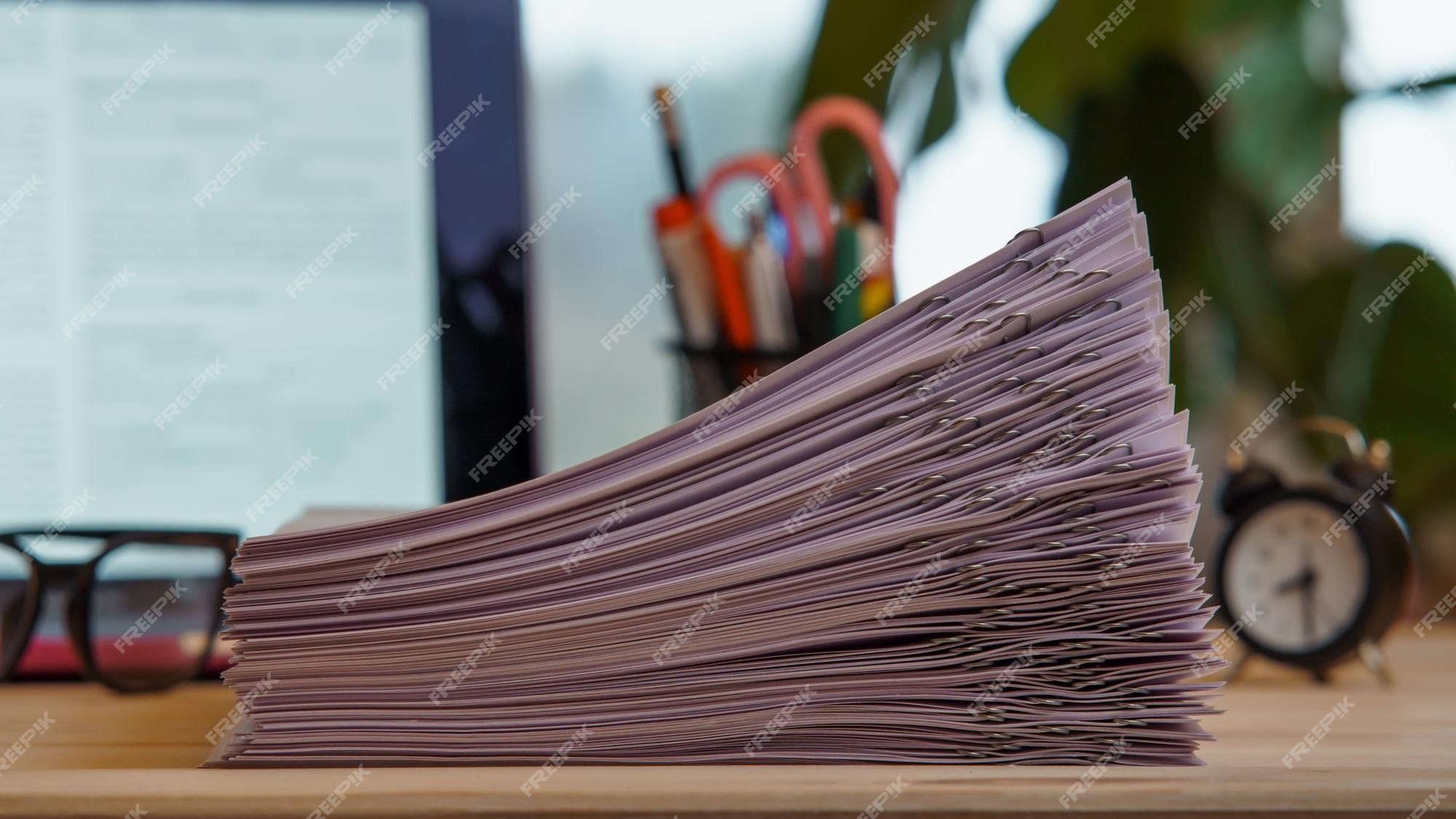This detailed photograph depicts a close-up of a desk scene, primarily showcasing a substantial stack of purple papers, estimated to be between 50 to 60 sheets thick. The right side of the pile is notably higher due to identical placement of paper clips on each document, creating a slant from approximately four inches on the right to two inches on the left. The setup suggests these could be graded tests or classroom assignments, awaiting distribution.

The stack rests on a brown, tiled ledge, against a blurred, well-lit background hinting at a classroom or office setting. Prominently visible in the background is a black cup brimming with various stationery items, including pens, pencils, scissors, highlighters, and magic markers. To the right, there's an old-fashioned alarm clock with a white face and black body, complete with little legs and bells on top. On the lower left, a pair of black glasses is visible. The overall scene is bathed in daylight, hinted by the brightness and possible presence of windows, adding to the clarity and vividness of the image. Additional elements include a computer or tablet screen, and the hint of a green plant, further enriching the context of this well-organized, academic or professional workspace.